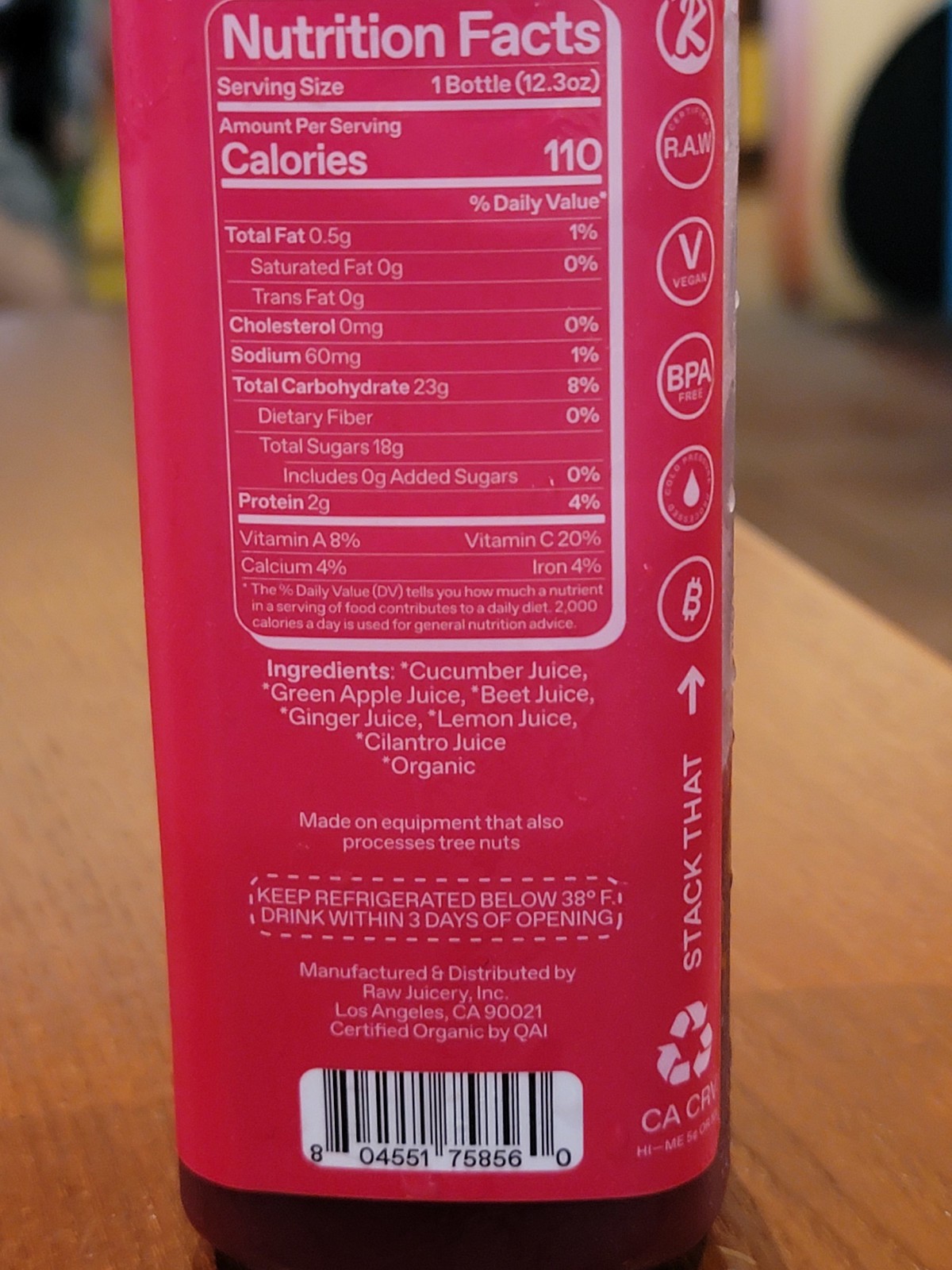This highly detailed close-up image showcases the nutritional facts panel on the side of a plastic juice bottle with a distinct red label. The nutrition facts panel, outlined in white and written in white text, prominently displays the serving size of one bottle (12.3 ounces). The detailed nutrition information includes 110 calories, 0.5 grams of total fat, 0 mg of cholesterol, 60 mg of sodium, 23 grams of total carbohydrates, and 2 grams of protein. Below the nutrition facts, we find the ingredients listed: cucumber juice, green apple juice, beet juice, ginger juice, lemon juice, cilantro juice, and the term "organic." Additional notes indicate that the juice is made on equipment that also processes tree nuts, and it features a dashed-bordered rectangle advising to keep the beverage refrigerated below 38 degrees Fahrenheit and to drink within three days of opening. 

Near the bottom of the label, it states "manufactured and distributed by" alongside a large barcode located at the bottom right corner. Vertically aligned logos run down the side, including circular symbols with an 'R,' 'raw,' 'V1,' 'BPA-Free,' a water drop icon, an arrow pointing up with the word 'stack,' and a recycling symbol. The scene is set on a natural-colored wood grain table, slightly out of focus to highlight the bottle, which appears to contain a brownish liquid.